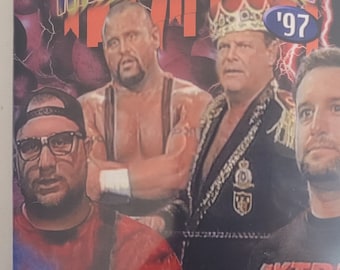This image appears to be an old, faded magazine cover or possibly a VHS/DVD cover from 1997, evident from the '97' marked in a small purple oval in the upper-right corner. The scene features four men, likely wrestlers based on their physiques and attire, arranged in a tiered formation.

At the back and slightly elevated, the most prominent figures are two muscular wrestlers. On the right, a mature man dons a regal outfit with a black robe, gold trim, and a king's crown, resembling a royal persona. He goes shirtless. Adjacent to him, another imposing wrestler has a shaved head and goatee. He's wearing spandex overall-style suspenders, no shirt, and has his wrists wrapped, posing with his hands crossed against a broad, oily chest.

In the front corners, two figures likely serve as commentators or supporting characters. On the left, a man with light facial hair, glasses, and a backwards baseball cap evokes a nerdier image, sporting a tie-dye shirt. On the right, there stands an average-looking man with short brown hair, wearing a black graphic t-shirt. This detailed composition suggests a dynamic and iconic representation of wrestling entertainment from the late '90s.